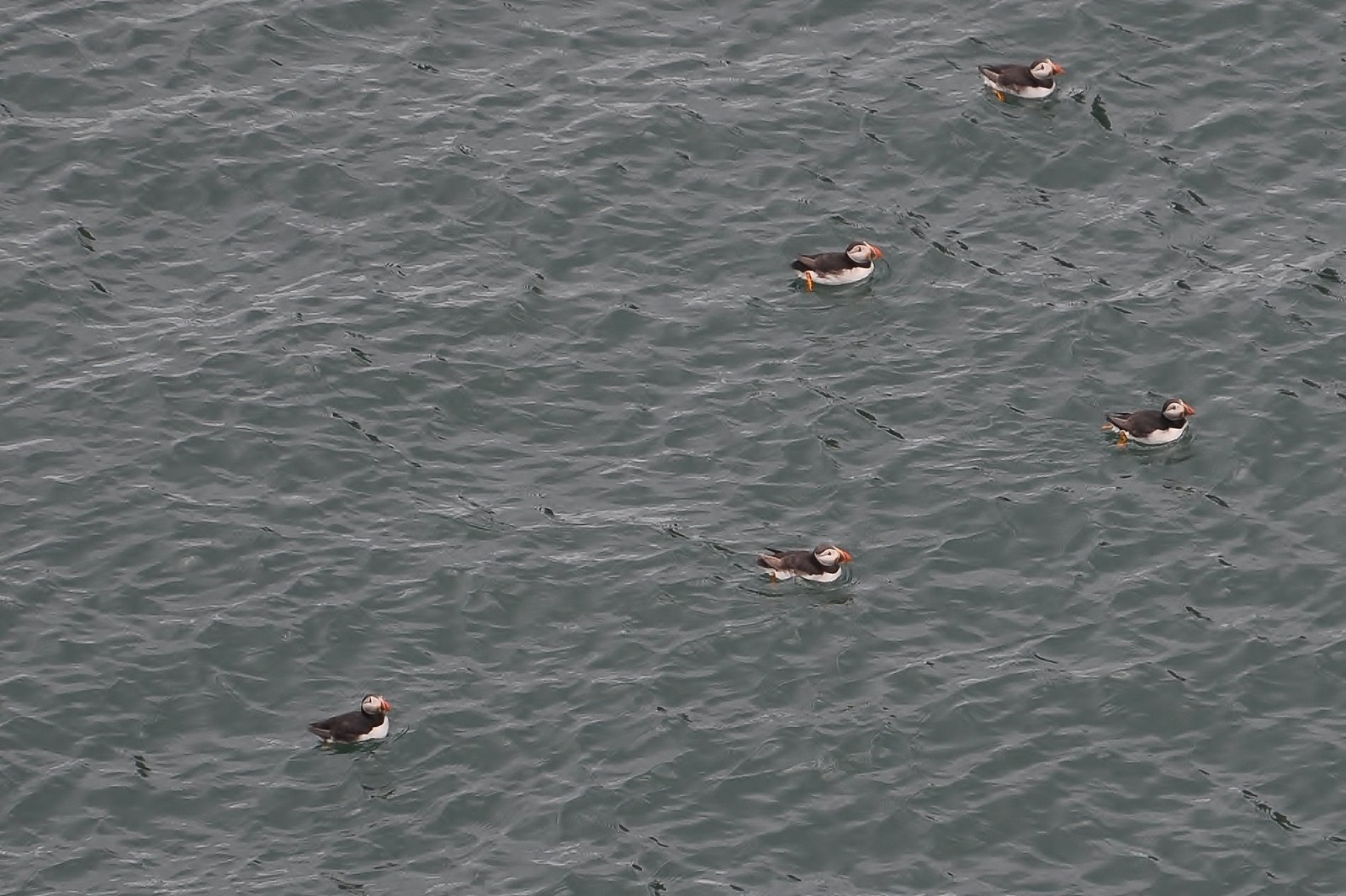In this image, we are looking down at a scene involving five ducks swimming in a large, somewhat dark and textured body of water, possibly located in the mid-Atlantic or northeastern region. The ducks, which have distinctive orange beaks, white faces with black eyes, and black feathers along their backs, are dispersed but all moving in the same direction. One duck, positioned slightly apart from the others, is glancing upwards towards the camera, while the rest are swimming diagonally to the right. The water around them is slightly wavy, with noticeable waves trailing behind the ducks. Their orange webbed feet can be seen paddling just beneath the water's surface. Despite appearing small in the photo, likely around an inch in length, these ducks are undoubtedly larger in real life.